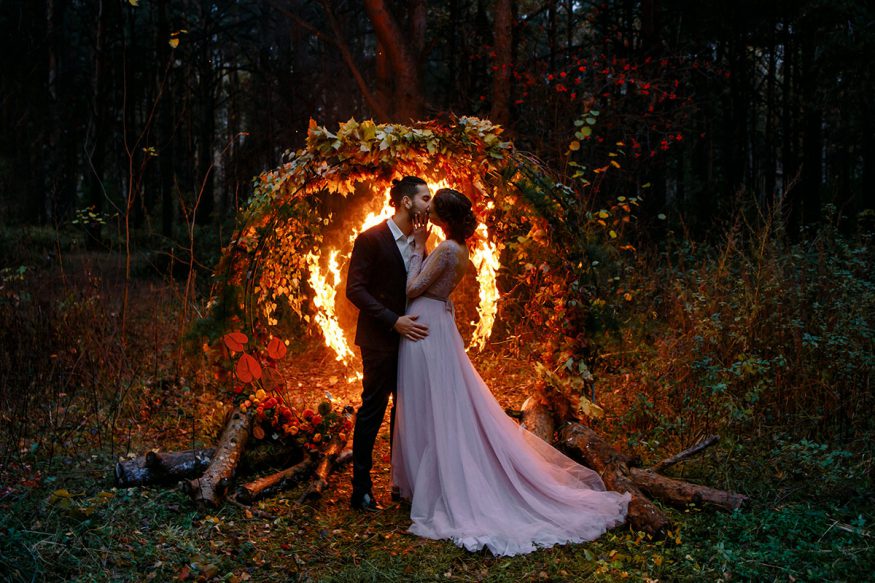In this captivating and adventurous wedding photograph, a young couple is immersed in a romantic photoshoot set in the heart of a dense forest at dusk. The natural surroundings feature trees, grass, and logs, creating a serene yet rustic atmosphere. The bride is elegantly adorned in a long, trailing white gown with lace detailing and a belt at the waist, though the lighting gives it a subtle pink hue. Her groom dons a black suit and white shirt, emphasizing a classic, timeless look. Against the backdrop lies a meticulously arranged circular structure made of vines, branches, and flowers, with a striking circle of burning fire within it, creating a dramatic and enchanting focal point. The couple shares a tender kiss in front of this fire, their silhouetted forms beautifully illuminated by the flames. Despite the ethereal and mesmerizing setting, the proximity to the fire adds an element of daring to this memorable and picturesque moment.